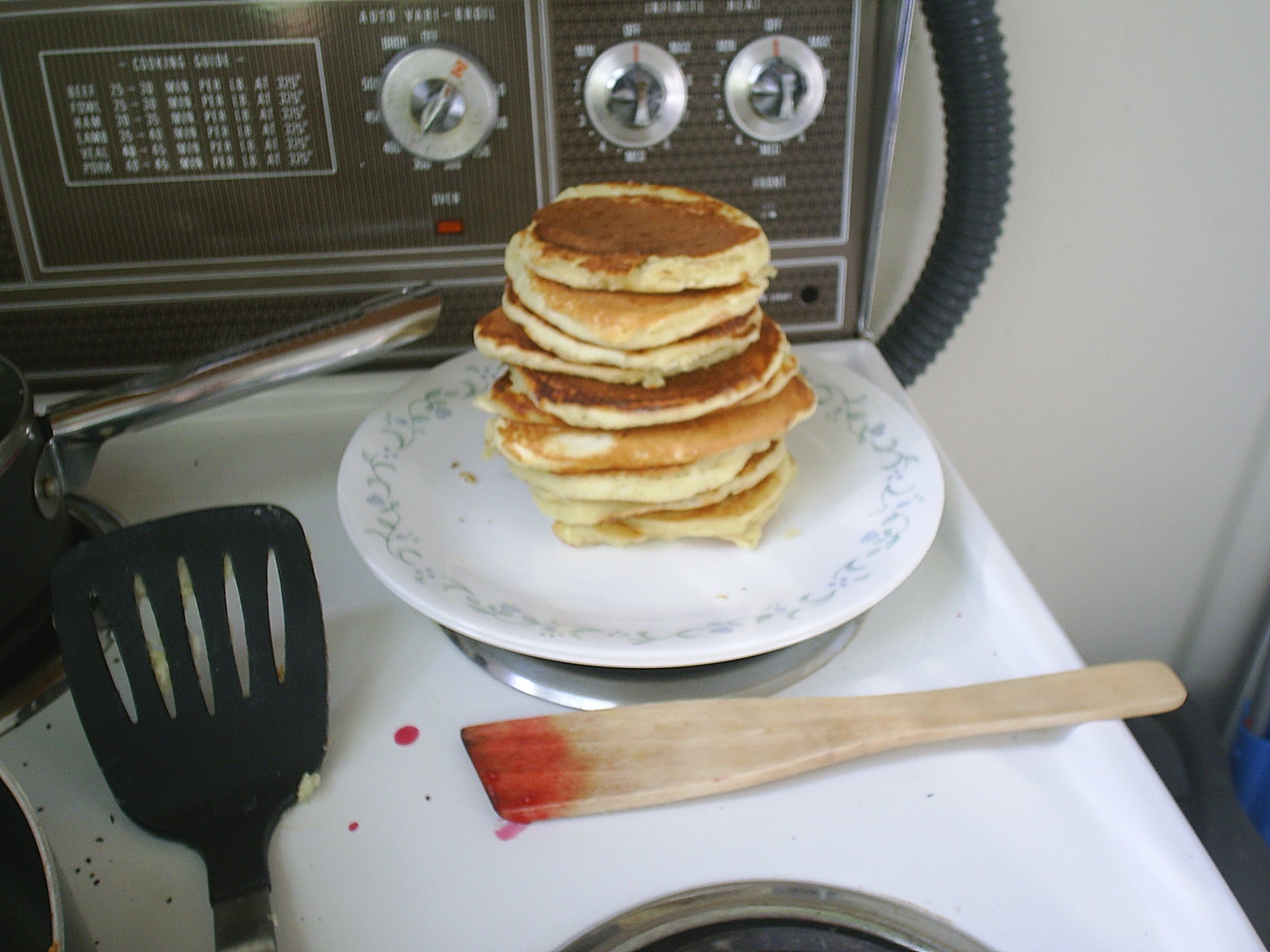This slightly blurry and somewhat out-of-focus color photograph, likely taken with a digital camera or phone using a flash, captures a close-up view of a white retro stove with distinct metal accents and silver knobs, characteristic of a design possibly from the 1950s. The white stovetop features a metal-bordered iron burner, partially visible along with a dark-hued pot in the upper left. In the center of the image sits a small white ceramic plate with a subtle leafy floral pattern around the edge, holding a stack of small pancakes. In the foreground, a wooden spatula coated with a pinkish-red substance lies flat, while a black plastic spatula with possible pancake remnants is positioned to the left. The zoomed-in perspective reveals minor dirt marks and ink patches on the stove, and the blurry background shows more details, including the stove's brown-patterned backdrop and a partial view of the wall to the right, emphasizing the kitchen setting's rustic charm.